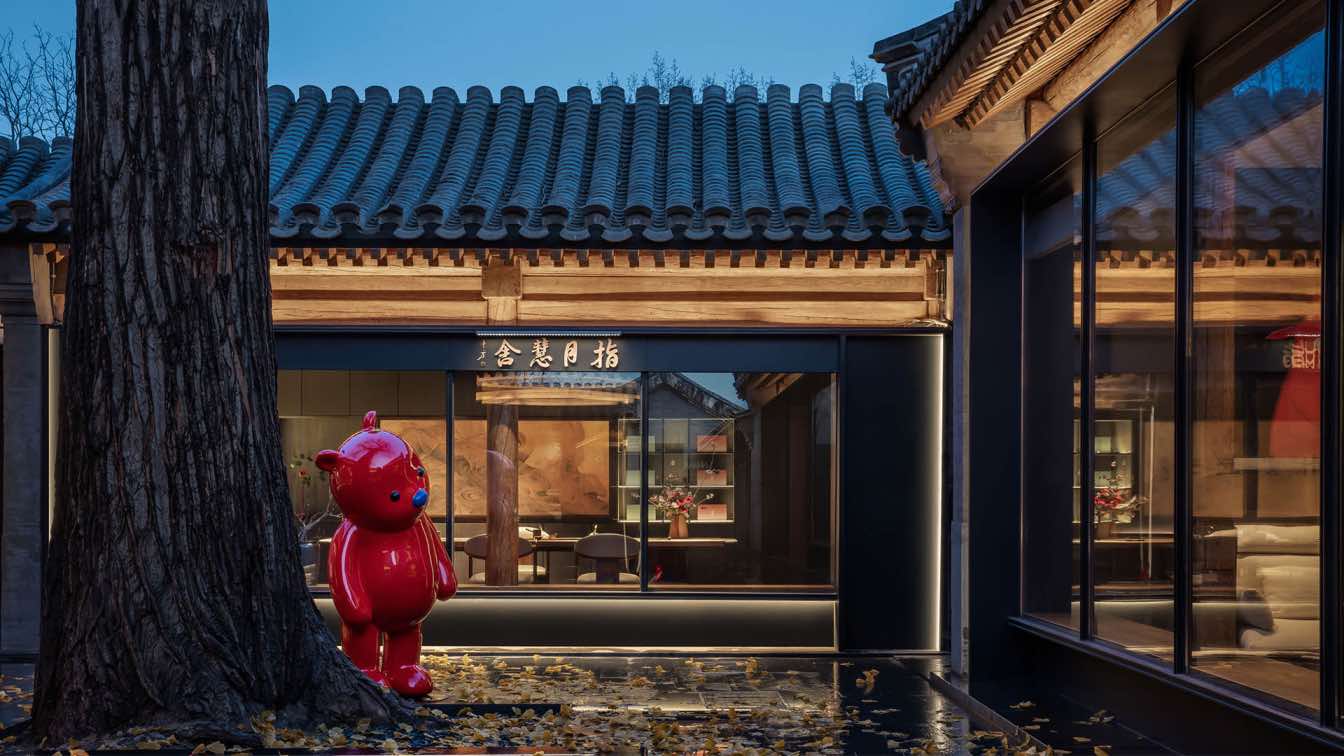The photograph, captured in the evening, presents a detailed view of an outdoor courtyard, showcasing two buildings. The image is rectangular, measuring approximately 6 inches wide and 3 inches high. Positioned to the left and directly ahead, the buildings feature large, reflective windows that mirror the outdoor environment. The rooftops are adorned with black tiles, transitioning into eaves made of light brown wood. The building in front displays a sign with golden Asian lettering, indicating a possible fine dining restaurant in China or Japan. Below a massive brown tree trunk situated to the left, there's a glossy red statue of a bear with its head tilted, seemingly peering into the right-hand building's windows. The exterior is accentuated by an ornate wood grain above the windows. The ground outside is granite-like, and the sky above is a deep blue with a slight highlight, suggesting late evening or dusk. Inside the front building, visible through the windows, are beige chairs, a table with a bouquet of flowers, and white shelves. The photograph is vibrant and clear, perfectly capturing the serene and meticulously detailed courtyard setting.